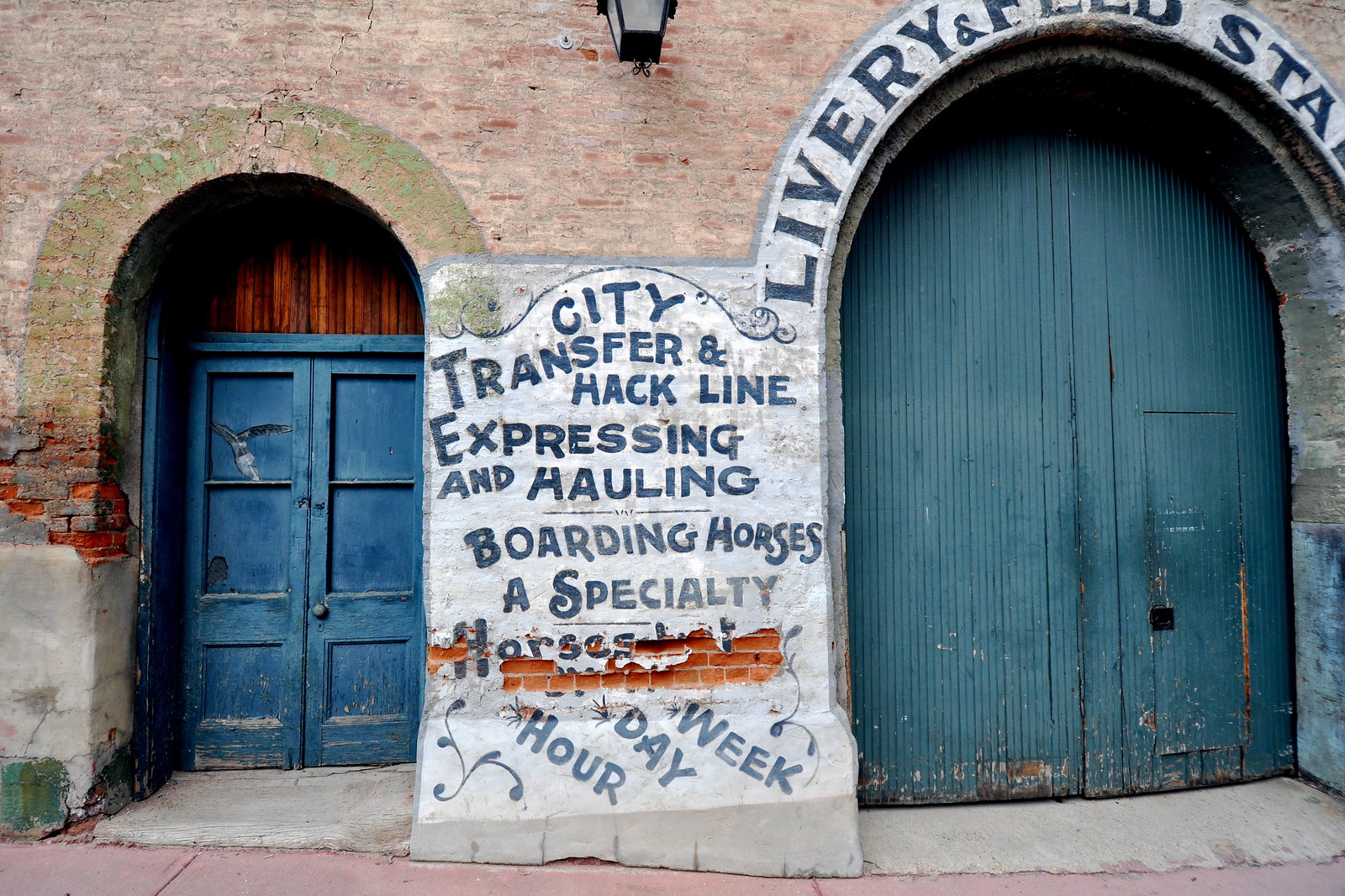The image depicts the exterior of an old, weathered building, possibly a warehouse, viewed from the sidewalk. The building's facade is made of aged, crumbling brick that has been painted over, and features two arched doorways. The door on the left is a smaller, wooden man door, painted blue, with signs of wear like fading and small cracks. To the right, there is a larger, taller blue wooden door, also showing signs of aging, and possibly large enough for vehicle entry, hinting at its use for deliveries. Between the two arches, a vintage lamp hangs above a faded, painted sign on the wall that reads, "City Transfer and Hackline Expressing and Hauling Boarding Horses as Specialty Horses. Our Day Week.” Above the right-side door, additional text reads "Library and Feed Stable." The ground in front of the doors is gray concrete, and the street in front is a faded pink color, adding to the overall sense of historical charm and decay.